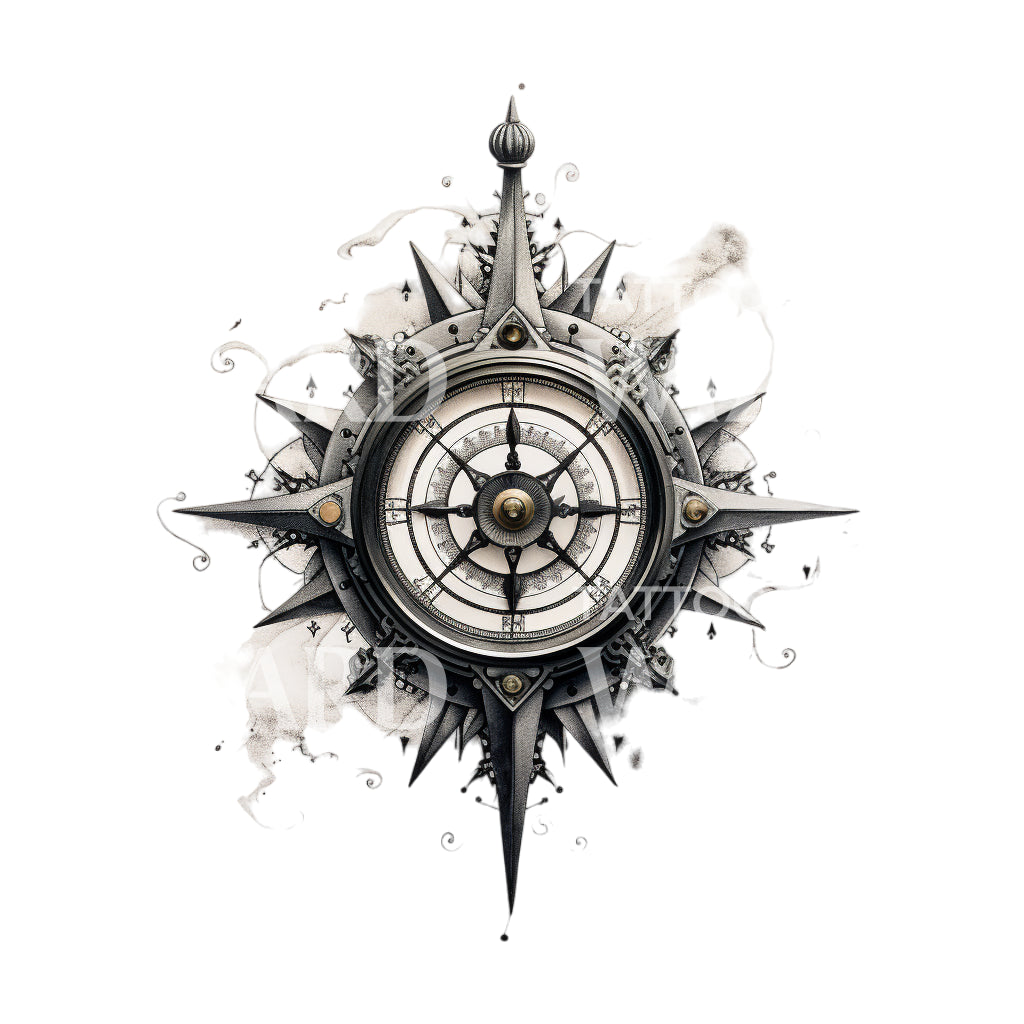The image is a detailed color illustration, predominantly black and white with subtle touches of brown and gray, resembling a steampunk fantasy compass. Despite its intricate design, it lacks the traditional north, south, east, and west indicators. The compass has a round face with multiple points extending outward, appearing ornate and spiky. A finial at the top resembles a wind turbine or an onion dome from Russian architecture, adding to its fantastical element. The bottom spike looks akin to the blade of a sword. The background portrays a snowy landscape, enhancing the ethereal appeal of the piece. Across the top, a faint watermark, likely reading "Tattoo," suggests that this could be a potential tattoo design. The compass's rustic metal appearance, combined with decorative spikes and ribbon-like elements, encapsulates a fusion of futuristic and fantastical aesthetics.